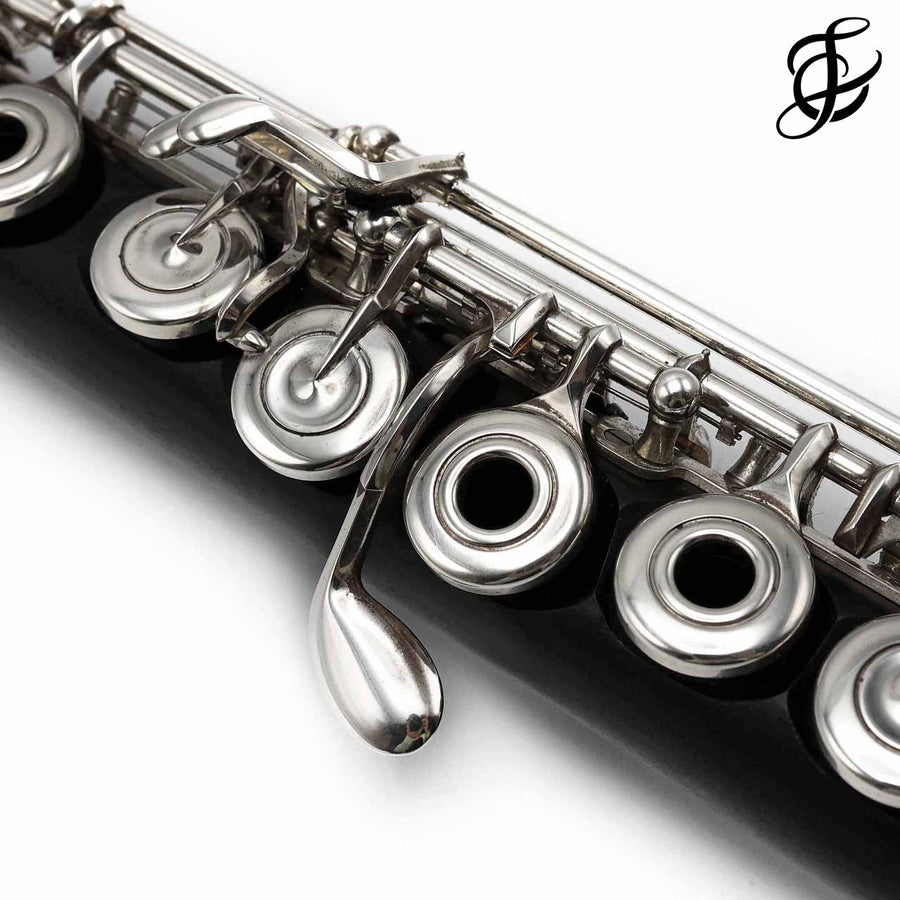This image depicts a close-up of what is likely a wind instrument, possibly a clarinet or perhaps an oboe. The instrument displays a sleek, chrome-like metallic frame with several keys visible. The keys, designed for finger placement to manipulate sound, exhibit a shiny, polished finish. The instrument features both metallic and black elements, with the black section appearing around the horn area, though the bell is not visible in the image. The background is entirely white, enhancing the clarity of the instrument details, and there is a logo in the upper right corner that looks like "LC". The clean, minimalist setting focuses attention on the intricate design and functionality of the wind instrument.